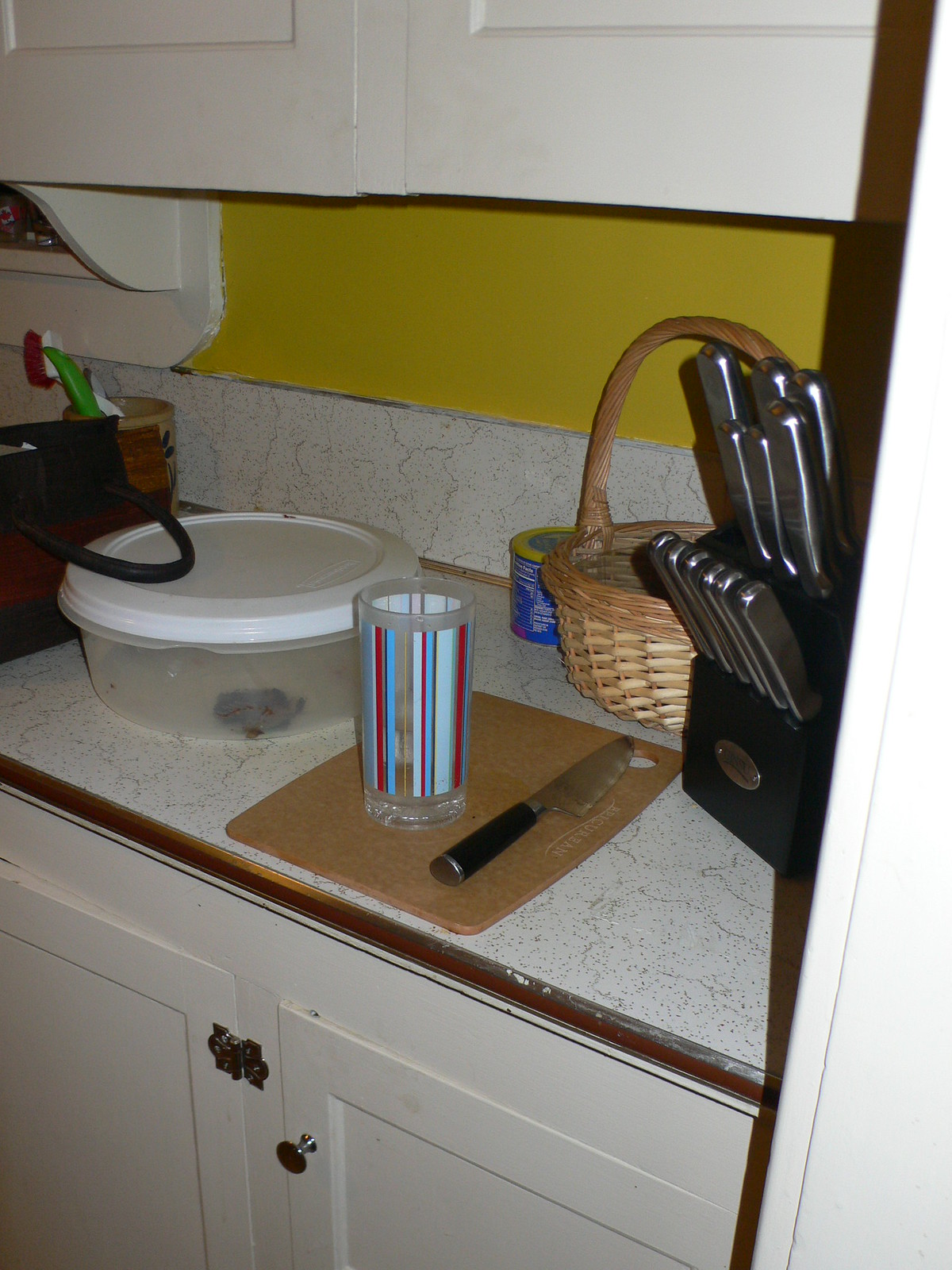A nostalgic snapshot of an antiquated kitchen counter in an older home captures the essence of time gone by. The counter is topped with a classic white Formica surface adorned with a faux marble pattern, encased by a worn wooden laminated edge that bears the marks of years of use, including visible chips. This vintage counter rests on white cabinets with aged hardware featuring silver hinges and knobs; the cabinet doors below show signs of misalignment, further reflecting their long service.

Running along the back of the counter is a six-inch high backsplash, mirroring the white Formica with gray marbling, extending to the base of a window peeking out from the left corner of the image. Above the backsplash, the kitchen wall is painted a dated mustard yellow, enhancing the vintage atmosphere. The lower parts of upper cabinets are visible, adding to the enclosed, cozy feel of the kitchen space.

To the right of the scene is a set of knives in a holder with sleek silver handles, suggesting a touch of modernity amidst the retro setting. Beside the knife set sits an empty wicker basket, and next to it, a small blue can with a yellow lid resembling a coffee canister. In front of the basket, a cutting board places prominently, holding both a knife and an old-fashioned glass with vertical red and blue stripes.

On the left side of the cutting board, a Tupperware container with a white plastic lid holds a single dark brown item, possibly a cookie or a brownie. Beside that, a bamboo-style container holds dish scrub brushes, followed by a small bag with an obscure content, identifiable only by its looped handle.

This detailed composition not only portrays the physical attributes of the kitchen but also evokes a sense of history and homeliness, reflecting the enduring legacy of an older home's heart and soul.